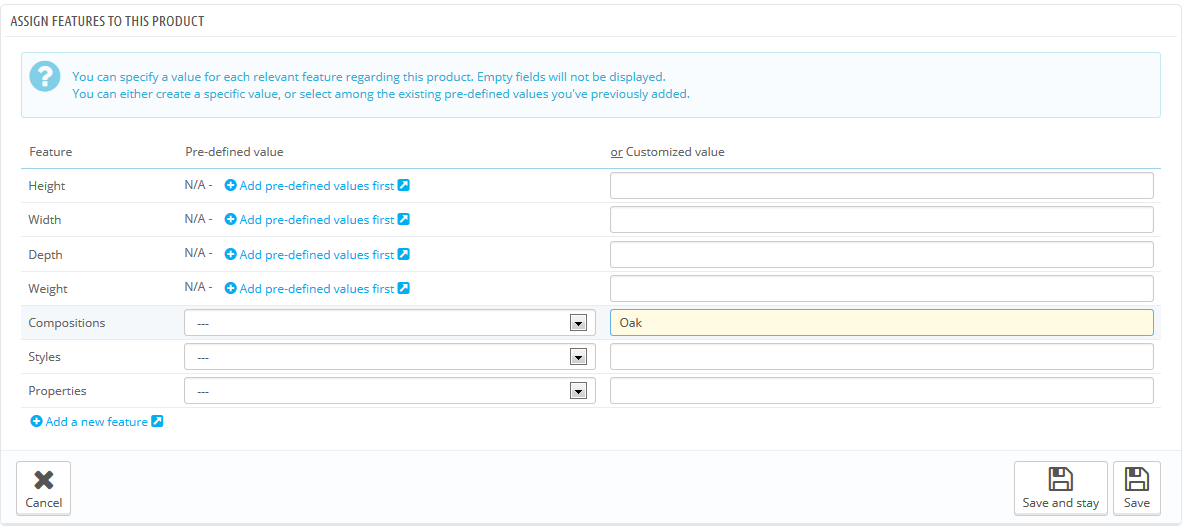This product configuration interface allows users to assign specific values to relevant features of the product. Users can input values for various features such as Height, Width, Depth, Weight, Composition, Style, and Properties. Each feature can have a custom value or a predefined value selected from a list that users have added previously. A designated field is available for entering custom values, while predefined values must be added first if they are to be used.

The Composition feature has been tagged with a custom value of "Oak," rather than a predefined value. The interface includes buttons for user actions at the bottom left, including a "Cancel" button marked with an X, a "Save and Stay" button, and a simple "Save" button. These buttons enable users to cancel their changes or save them while continuing to work on or leaving the interface. The icon used to denote saving data resembles an old hard disk, reinforcing the save function. The predominant colors of the interface are blue, white, yellow, and black.